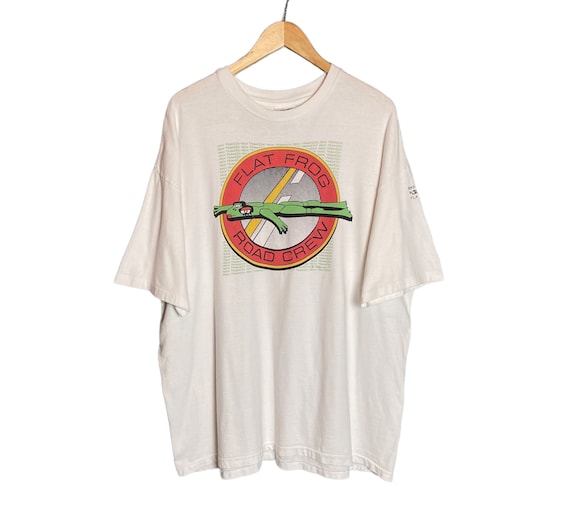This color photograph captures a white, baggy t-shirt hanging from a brown wooden hanger, photographed against a plain white background. The metal hook of the hanger is visible at the top. The t-shirt features a prominent graphic centered on the chest. The graphic is a red circle with a gold and black border. The black text within the circle reads "Flat Frog" at the top and "Road Crew" at the bottom. Inside the circle, a green, humanoid cartoon frog is sprawled out, resembling a flattened state, with red eyelids and red lipstick. The background within the circle shows a depiction of highway pavement, complete with yellow and white diagonal stripes representing road markings. The graphic's pavement texture resembles a whiteish-gray pattern with divots, akin to a golf ball's surface. Overall, the image emphasizes the t-shirt's unique and playful design.